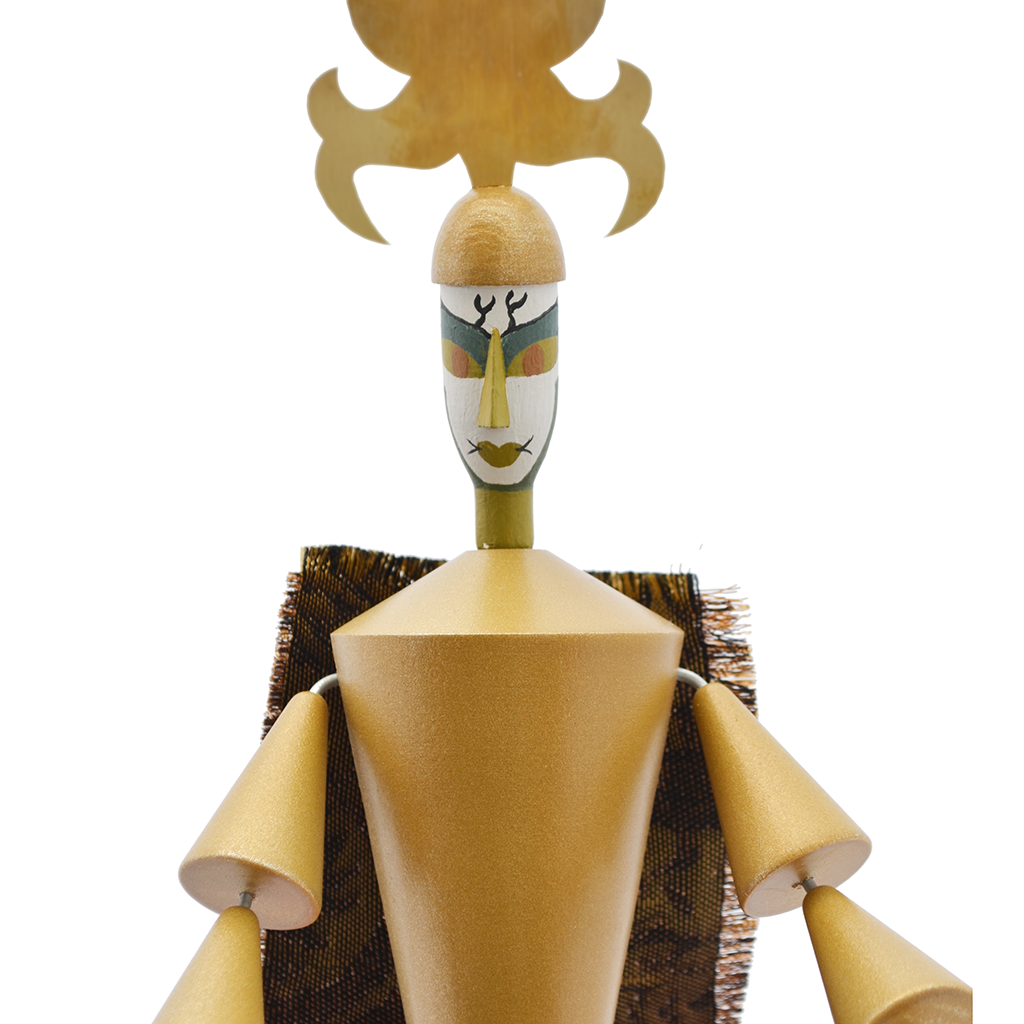The image depicts an intricately crafted wooden puppet-like sculpture. The figure's body appears to be designed in the shape of an upside-down Christmas tree, emphasizing a triangular structure. Made from light brown wood, the arms consist of stacked wooden cones, threaded together, resembling the shapes of trees. Although the hands are not visible, the attention to the unique arm construction stands out. 

The head of the puppet is fashioned from a wooden dowel, painted white, giving it a distinguishable, bright appearance. With orange and yellow eyes lined with green and black, the puppet conveys a curious and striking facial expression. It also features a pointy, square nose and well-defined lips. Above its painted face, the puppet wears a very decorative, flowery hat, crafted from the same light wooden material, adding a whimsical touch to its character. 

The background displays a white setting, providing excellent brightness and clarity to the image. Behind the figure, a dark brown fabric with fringes can be noted, enhancing the overall detail and texture of the backdrop, making the wooden figure stand out even more vividly.